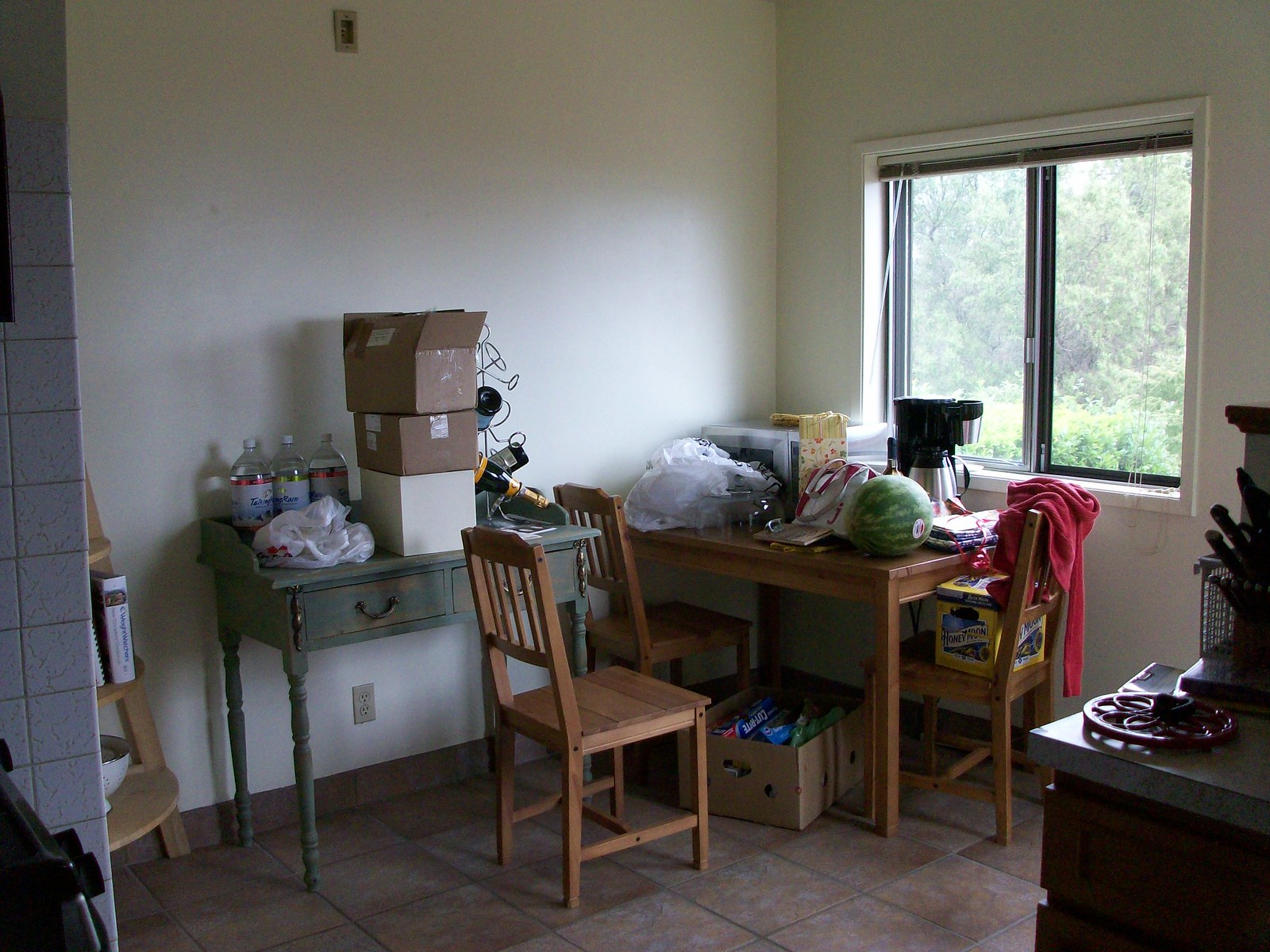This image showcases a cluttered storage room bathed in daylight. The focal point is a wooden table situated in front of a double-pane window with raised blinds, revealing a picturesque forest area outside. The table is strewn with an eclectic mix of items, including a coffee maker, a watermelon, various boxes, bags, and a red sweater. Accompanying the table are three wooden chairs, while beneath it lies another wooden box filled with miscellaneous junk.

To the left of the main table, there is a gray side table, equally cluttered, featuring three stacked boxes with wires spilling out, three plastic bottles, and additional plastic bags. The background features a white wall, contrasting with the brown laminate tile flooring.

On the right side of the image, a partial view of a counter emerges from the shadows. The counter appears equally disorganized, hosting items like a cutlery stand and what looks like the metal frame of a wheel. Overall, the room presents a chaotic and cluttered scene with various tables and miscellaneous items scattered throughout.